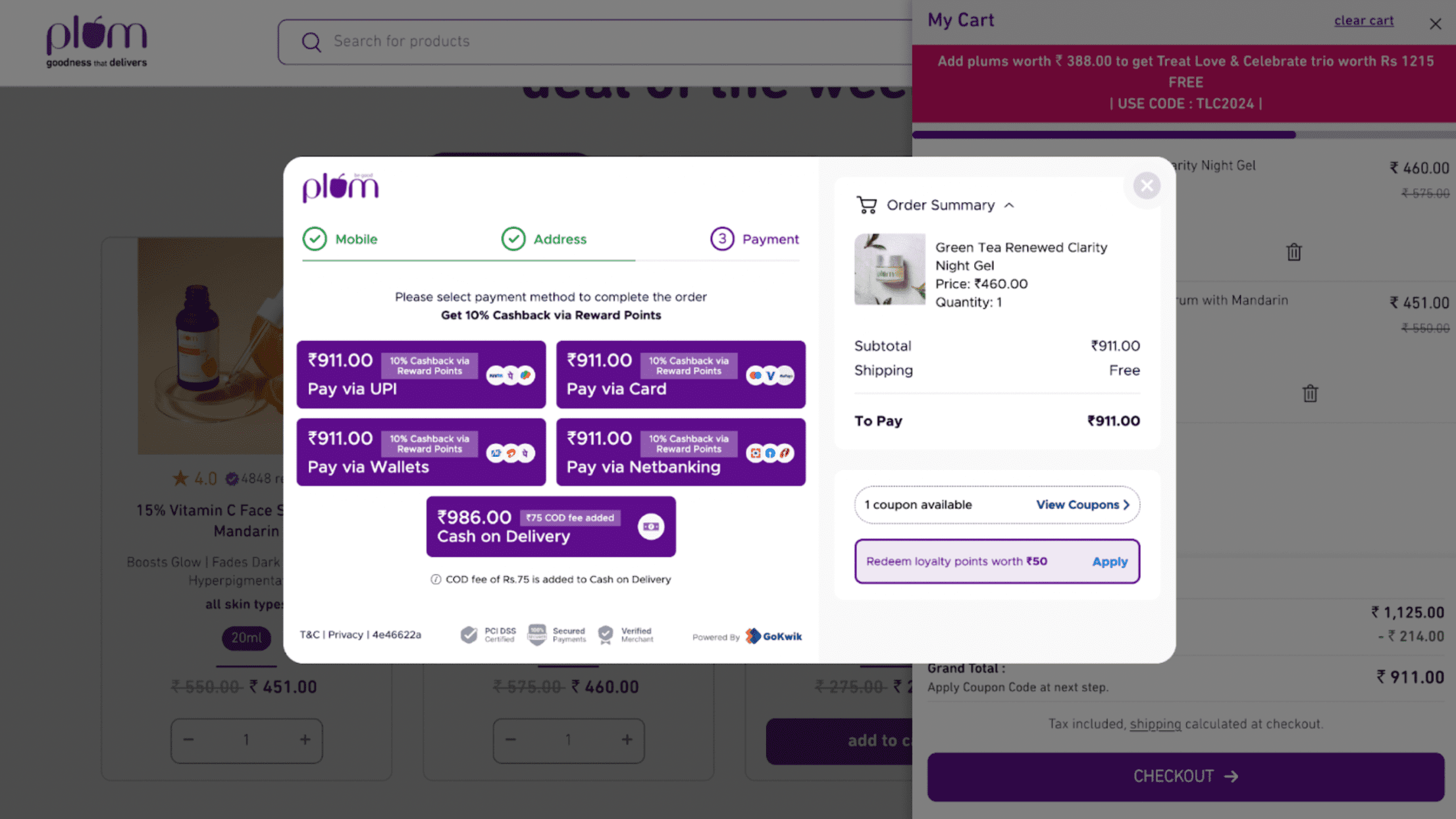An online shopping website interface is depicted, branded with the name "Plum" (abbreviated as "PL"). The page prominently features an image of a plum, followed by the letter "M." To the right of the screen are interactive options, including "My Cart," "Clear Cart," and an "X" button to close the cart. 

At the bottom of the interface, there is a section with additional information, partially overlaid by a pop-up window. The pop-up includes stages of checkout such as "Mobile," "Address," and "Payment," each accompanied by a checkmark, and is labeled with the number "3," indicating the current step in the checkout process. 

The order summary is visible within the pop-up, featuring an image and description of the selected product: "Green Tea Renewed Clarity Night Gel." The price is denoted by a Euro symbol and listed as €460. The quantity selected is 1, resulting in a subtotal of €460. There is no charge for shipping. The total amount is €460. The "Checkout" option is displayed at the bottom of the screen.